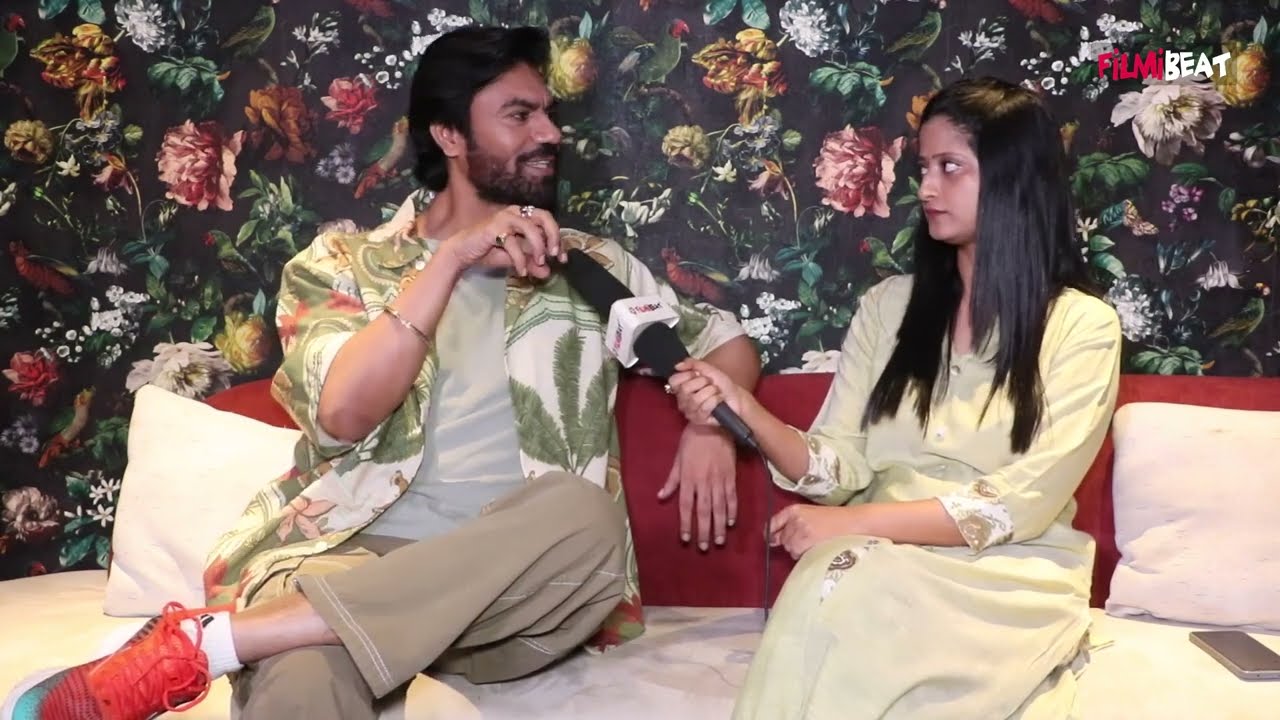The image depicts a man and a woman, both of Indian or Middle Eastern descent, seated on a red couch covered by a white sheet and adorned with two white pillows. The woman, with long black hair, wearing a beige dress, is holding a microphone while interviewing the man who is dressed in a vibrant floral shirt featuring white, green, and other colors. He is accessorized with two rings and a gold bracelet and is wearing striking red shoes. The man has black hair and a beard. Behind them, the wall features elaborate floral wallpaper with large flowers in pink, orange, yellow, and green, along with leaves and depictions of birds, including parrots. There is also text on the top right corner reading "Filmy Beat" suggesting a connection to an entertainment program possibly centered around films. A cell phone is visible next to the woman, possibly hinting at the interview being recorded or live-streamed.